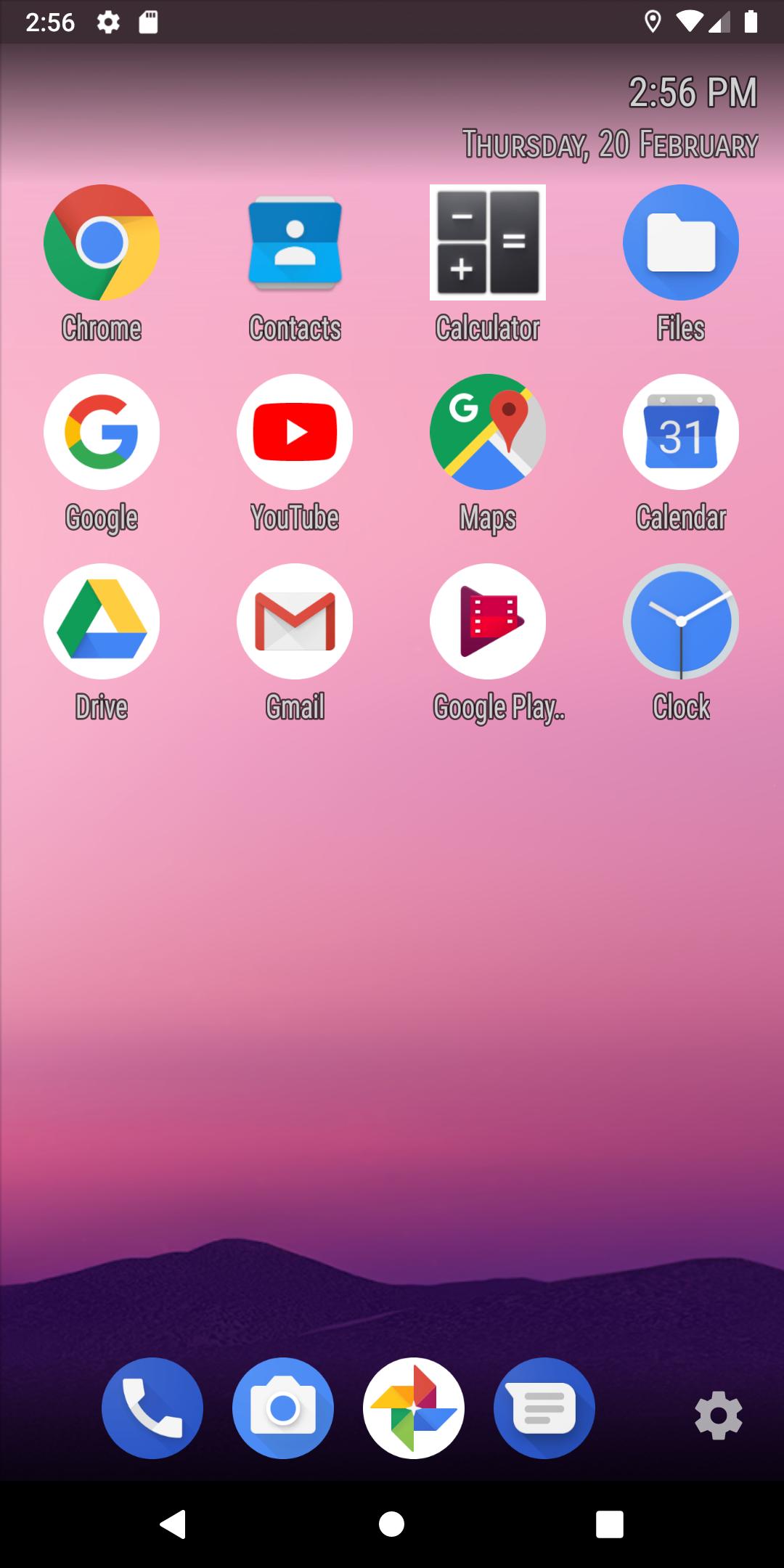Screenshot of a smartphone home screen displaying a vibrant, nature-themed wallpaper. The wallpaper features a gradient sky ranging from pink at the top to purple, transitioning above a silhouetted purple mountain. At the bottom of the screen, there's a black navigation bar with three icons: a back button, an open recent apps button, and a home button.

In the top left corner, the time is displayed as 2:56 p.m., along with icons for settings and a SIM card. The top right corner shows the Wi-Fi icon, half-filled data icon, and a full battery icon. The date, "Thursday, 20 February," is also displayed at the top right.

The main home screen is populated with various app icons, including Chrome, Contacts, Calculator, Files, Google, YouTube, Maps, Calendar, Drive, Gmail, Google Play, and Clock. At the bottom of the screen, there is a frequently-used apps dock featuring icons for Phone, Camera, Photos, Messages, and Settings.